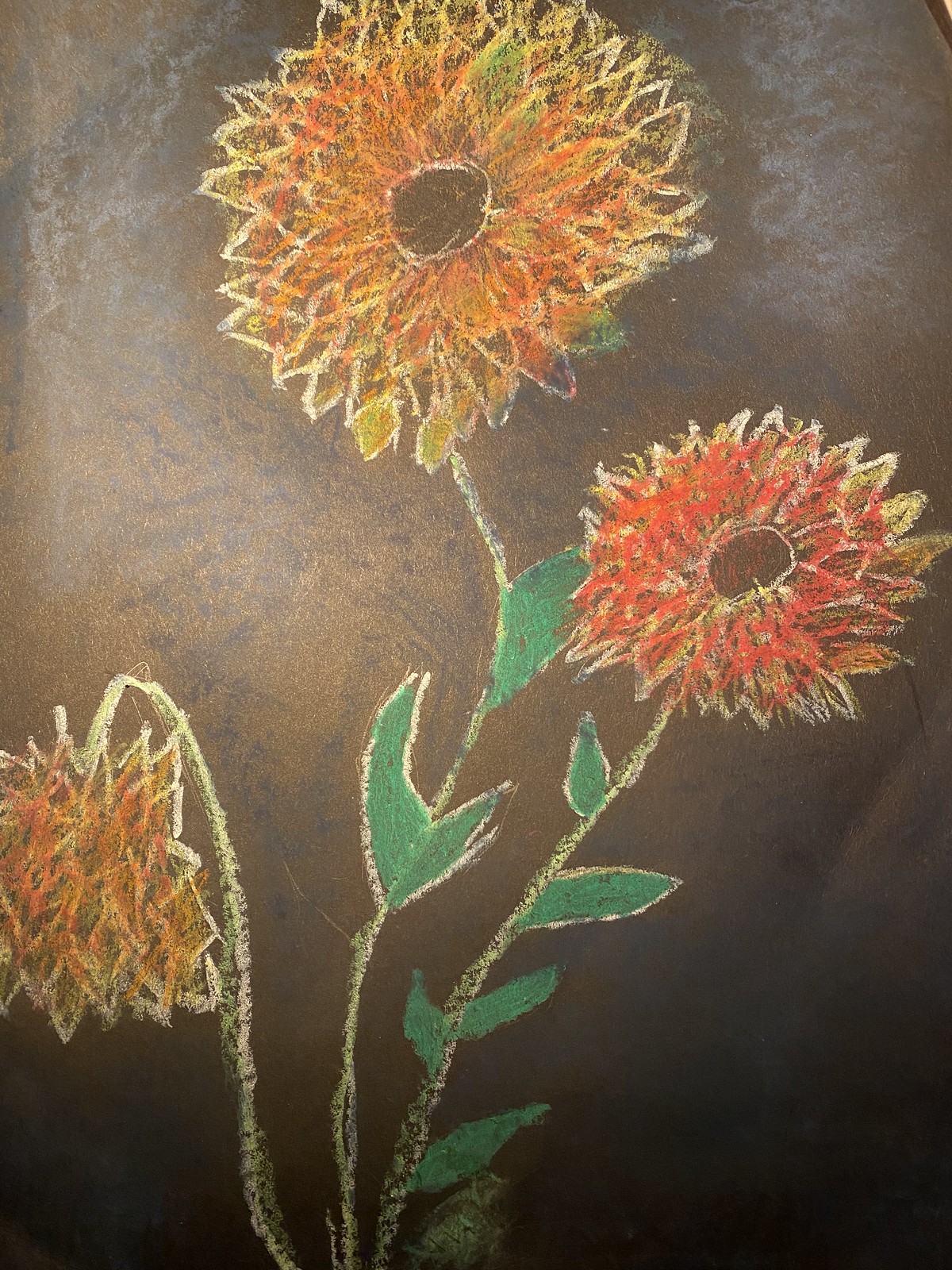This detailed color photograph showcases a chalk drawing on a weathered chalkboard with a black and brown, almost rusted appearance, possibly accented by a reddish tint. The art depicts three stylized flowers that span the entire height of the image, each with distinct features. The central flower, the tallest and largest, resembles a sunflower or daisy with vibrant orange, yellow, and red petals surrounding a dark, uncolored circular center. Its green stem is adorned with three leaves. To the right, a slightly smaller and more reddish flower of similar design has a stem with five green leaves and an undrawn circular center. The leftmost flower, slightly drooping, displays orange and yellow petals and lacks leaves on its stem. The chalk drawing incorporates subtle white highlights on the stems and petals, enhancing the visual depth, and hints at childlike simplicity. The photograph captures the reflective glare, likely from a camera flash, adding a shiny dimension to the chalkboard surface.